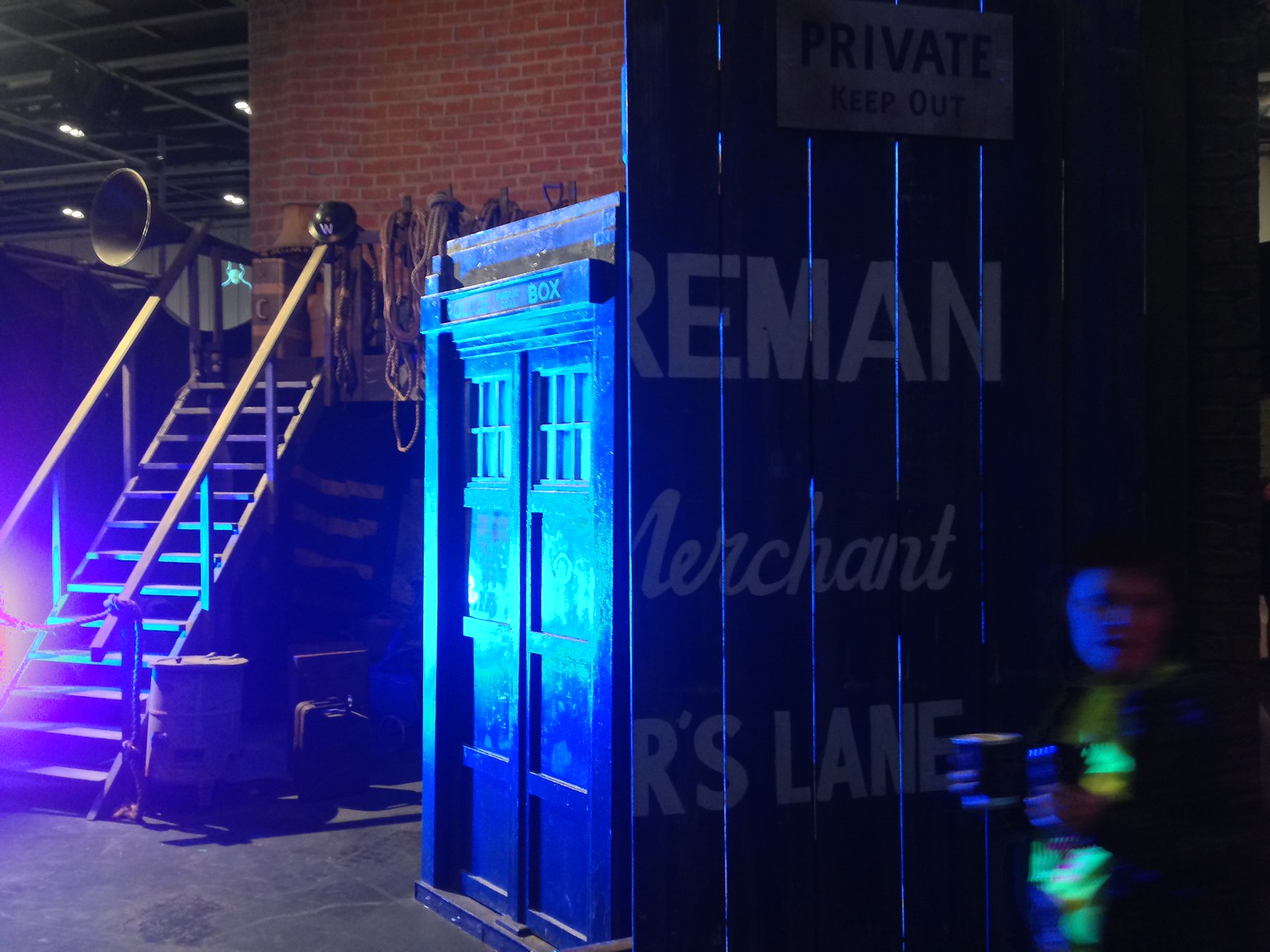In the image, a dark nighttime scene is captured featuring various elements suggestive of a themed venue or event. A prominent blue wooden box, resembling a British telephone booth, stands beside a red brick wall. The box, illuminated on its left side, sports vertical boards along its perimeter and two covered windows at the top. A white sign with dark letters reading "PRIVATE. KEEP OUT." is prominently displayed at its top. Below that, stencil-spray-painted text partially reveals the words "REMAN," "merchant," and "R'S Lane," though parts of these words are obscured. Adjacent to the box, a wooden staircase ascends directly into the brick wall, with rope barriers strung across its handrails at the bottom and various objects, including a bunch of ropes, hanging on the wall nearby. At the top of the stairs, a large, round loudspeaker extends over the wall, hinting at an industrial setting.

In the bottom right corner, an out-of-focus figure—a woman—holds what appear to be two cups, possibly beers, moving through the scene. Her shiny golden attire glimmers slightly in the dim light. In an apparent connection to a "Doctor Who" theme, the overall layout suggests an eventful and dynamically atmospheric setting. Bright yellow light spills from the bottom left corner, casting intriguing shadows on the blue box and the industrial elements around, such as a barrel near the base of the stairs, contributing to the overall mysterious ambiance of the image.